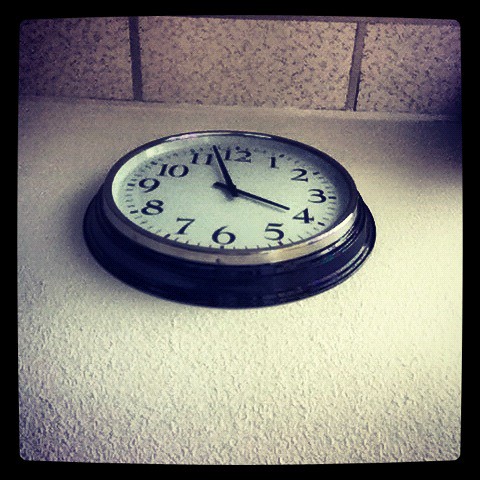The image depicts a clock mounted on a textured, creamy white wall, viewed from a low angle looking upward. You can see the white ceiling with gray grid tiles above. The clock is circular with a black outer rim and a silver-bordered face. It features black numerals from 1 to 12 and black hands. The face of the clock is white, and it's challenging to determine the exact time, as the hands appear similar in length, suggesting either 11:20 or 3:58. The aesthetic detail indicates the clock integrates seamlessly with its surroundings, blending modestly into the interior's subtle palette.